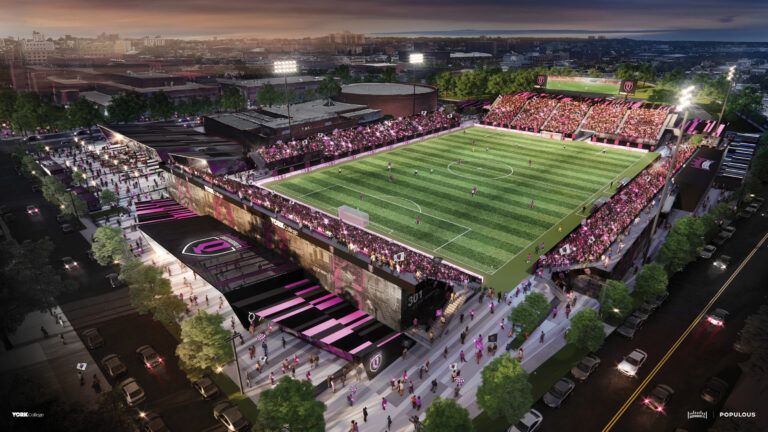The image is a detailed, virtual depiction of a large, outdoor soccer stadium captured in an overhead, landscape-oriented view, possibly created using a drone. The soccer field is characterized by alternating dark and light green horizontal stripes, with a circular white cutout at the center. Surrounding the rectangular field are stands filled with an audience, most of whom are dressed in the team's colors—purple and black. These colors are also evident in the team's insignia, a shield with a "Q", which is prominently displayed at the far end of the field and on a big black roof at the grand entrance on the left-hand side. The stadium is well-lit by four large stadium lights positioned along the long sides of the rectangle, with two on each side. Beyond the stadium, there is a generic cityscape, roads on both the left and right sides, and numerous people walking around, contributing to the bustling atmosphere.